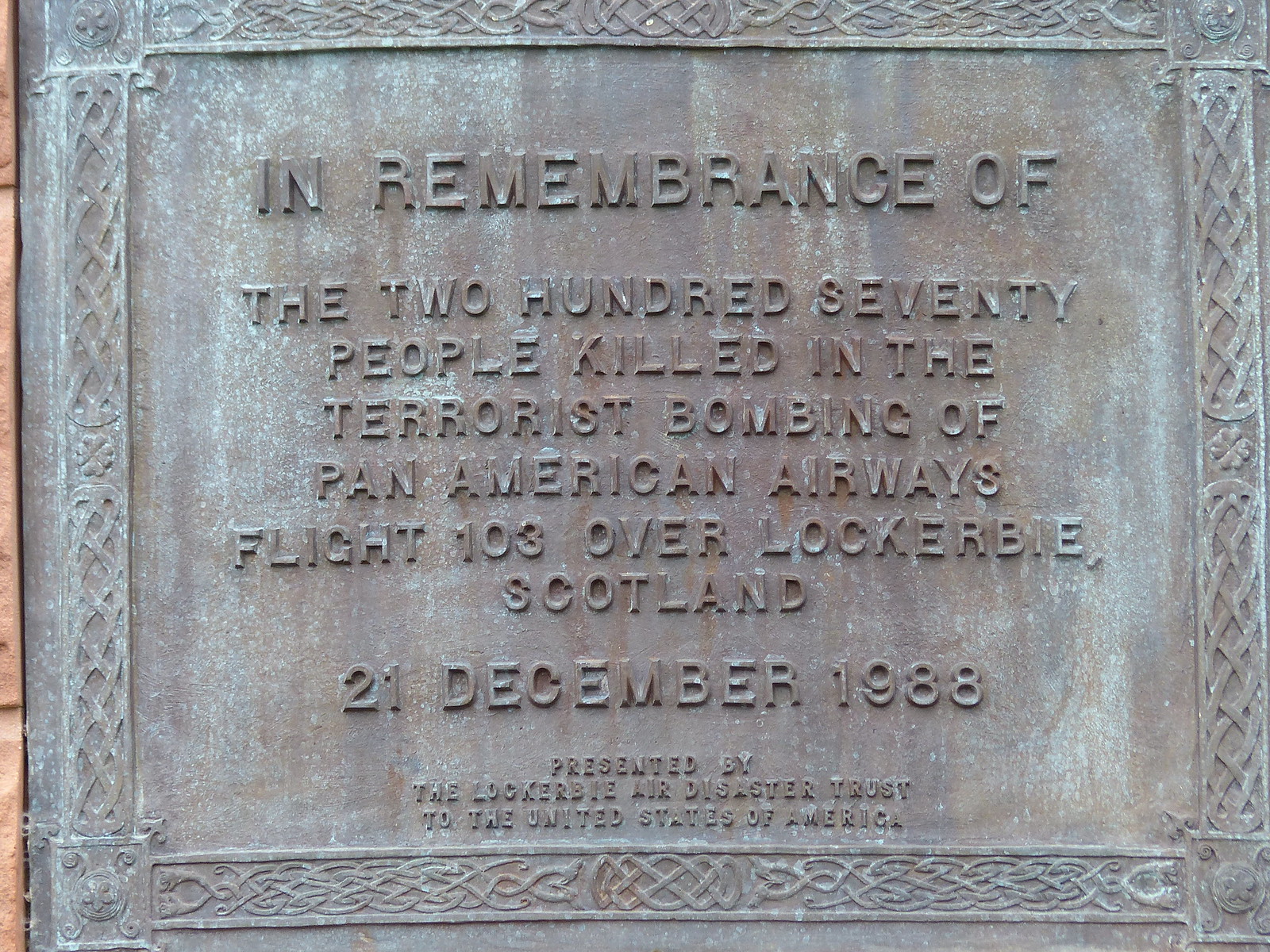This image depicts a weathered and aged outdoor memorial plaque commemorating the 270 victims of the terrorist bombing of Pan American Airways Flight 103 over Lockerbie, Scotland, on December 21, 1988. The plaque, presented by the Lockerbie Air Disaster Trust to the United States of America, features engraved text and a decorative border with an Irish motif, including four-leaf clovers. The material appears to be metal, showing signs of oxidation with a gray hue and patterned edges.